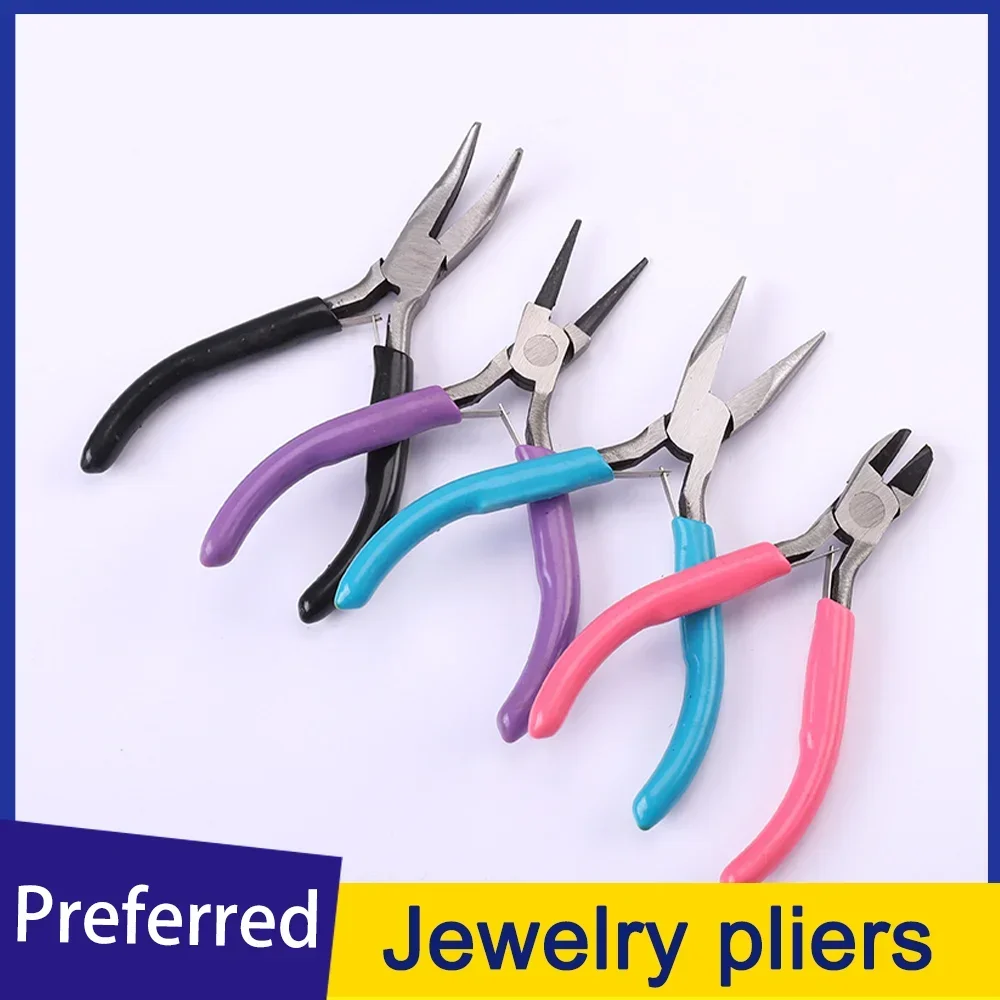The image features an advertisement for jewelry pliers, bordered by a small dark blue line around the top and sides, and a purple line that continues around except for the bottom right corner, which is overlapped by a yellow box. In the yellow box, the text "Jewelry Pliers" is written in a purple font. Below the image, in a purple box with white text, it reads "Preferred."

The background of the image is off-white, showcasing four pairs of jewelry pliers, each with a different colored handle, arranged diagonally with one leg crossing the handle of the next. From left to right, the handles are black, purple, blue, and pink. Each pair of pliers has a distinct metal top - the first has a large sharp part, the second has a smaller part, the third is wider, and the fourth is notably small. The overall appearance of the pliers varies slightly but they are all designed for jewelry work.